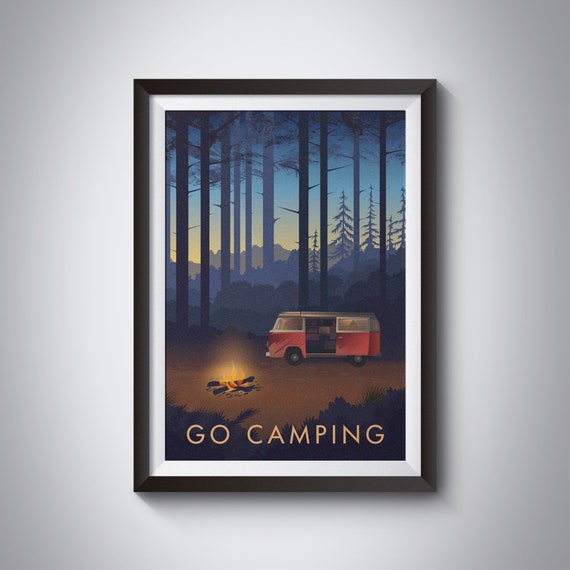The image depicts a framed poster hanging on a beige-painted wall. The poster is enclosed in a simple black frame with white matting. It features a painted illustration of an old-style red and white Volkswagen camper van, parked in a clearing in the woods during dusk, suggested by a hint of yellow in the sky. The van's side door is open, revealing a counter and table inside. To the right of the van, a small campfire is ablaze with logs crisscrossed at the base. Surrounding the scene are rows of very tall pine trees with foliage concentrated at the tops, and in the distant background, outlines of mountains and additional fir trees fade into a hazy blue. At the bottom of the poster, in large, plain font, the words "Go Camping" are prominently displayed. The illustration is characterized by its use of solid colors and minimalistic shapes, capturing the essence of a tranquil camping experience.